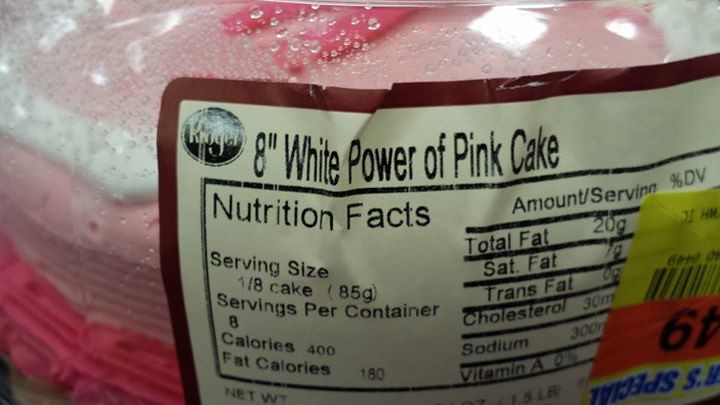In this horizontally oriented image, we are given a detailed view of a label affixed to a plastic-wrapped item. The label is attached to the corner of the packaging for a cake. Through the clear plastic, the cake is visible and features intricate decoration: pink frosting with white piping around the top, a lighter shade of pink in the center, and a darker pink adorning the sides near the bottom.

The label itself has a brown outline and a beige background with dark brown text. It prominently reads "Kroger 8-inch White Power of Pink Cake." Below this, nutritional information is provided, showcasing details like serving size, number of servings per container, calories, and fat calories. The overall presentation and the specific design of the label and cake create a visually appealing and informative display.